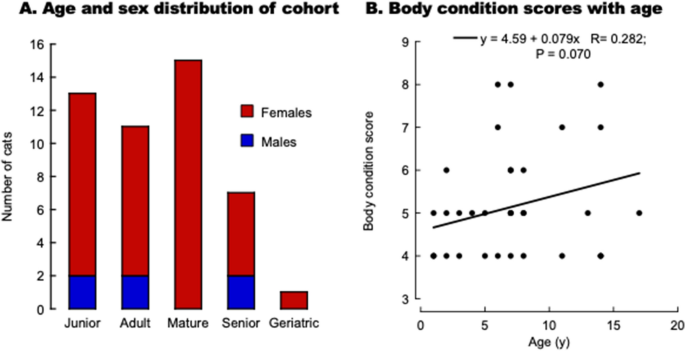The image displays two graphs side-by-side labeled A and B, offering a comprehensive visualization of demographic and physical condition data for a cohort of cats. 

**Graph A: Age and Sex Distribution of Cohort** is a bar graph with bars segmented into red and blue sections, representing female and male cats respectively. The y-axis, labeled "Number of Cats," ranges from 0 to 16. The x-axis categorizes the cats by age groups: Junior, Adult, Mature, Senior, and Geriatric. Notably, the number of females exceeds that of males in each category, with no males present in the Mature and Geriatric groups. Specifically, the counts are as follows: Junior (13), Adult (11), Mature (15), Senior (7), and Geriatric (1).

**Graph B: Body Condition Scores with Age** is a line graph populated with individual data points. The y-axis, labeled "Body Condition Score," ranges from 3 to 9, and the x-axis, labeled "Age in Years," spans from 0 to 20. The graph illustrates a general upward trend in body condition scores with age, depicted by a line going diagonally from just below 5 to about 6. The top of the graph includes a linear regression equation: y = 4.9 + 0.079x, with the correlation coefficient r = 0.282, and p-value = 0.070, suggesting a weak yet positive correlation between age and body condition scores. Most data points cluster around scores 4 and 5, although scores of 6, 7, and 8 are also represented.

Overall, these graphs provide detailed insights into the age, sex distribution, and physical condition of a specific cohort of cats, emphasizing a predominance of females and a slight trend of improved body condition with age.